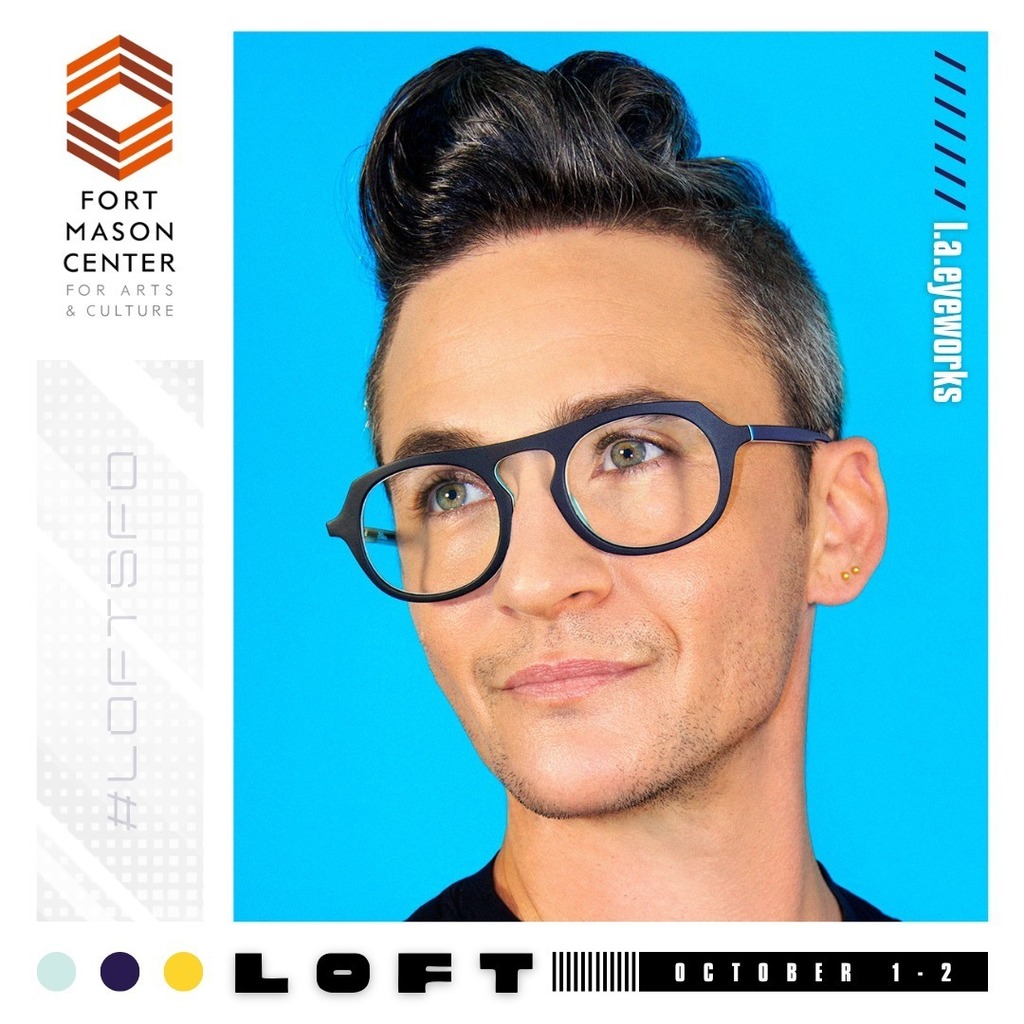The photograph is a detailed advertisement with a bright blue background, featuring a person with Caucasian skin and dark hair styled in a pompadour, with hints of gray at the temples. They wear striking dark blue eyeglasses and have hazel eyes accented by a light stubble on their cheeks, chin, and upper lip. The person is clad in a black shirt, with the photo cropped to show just the top of their shoulders. They are looking away from the camera to the left. On the left side of the image, there's a white strip with a logo featuring three upside-down red and orange V's, repeated in reverse, along with the text "Fort Mason Center for Arts and Culture" and "#LOFT SFO." At the bottom left, there is a sequence of a light blue dot, a dark blue dot, and a yellow dot, above the chunky text "LOFT" and "October 1-2" over a black strip. The top right corner features several slanted dark blue lines with the text “L.A.I.Works.” The ad appears to promote eyeglasses, with the combination of visual elements drawing attention effectively.